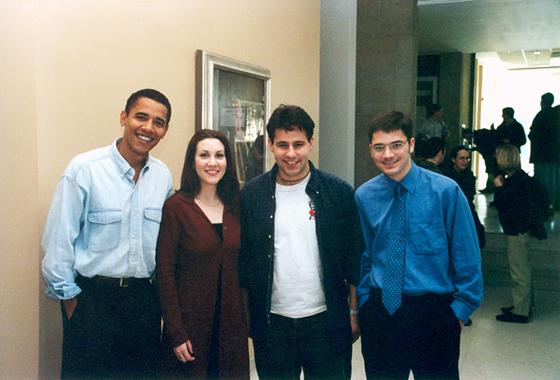In this horizontally oriented, realistic photograph, a young Barack Obama is captured in what appears to be a dimly lit hotel lobby or a similar interior setting, alongside three other individuals. The beige floor and yellow walls are complemented by a gray column on the right side, and an indistinct group of people can be seen in the poorly lit background. Central to the image are Barack and his companions, presumably at a casual or networking event. Barack, smiling with his hands in his pockets, wears a light denim shirt and black slacks. To his right is a fair-complexioned woman with long, straight black hair, dressed in a maroon sweater dress over a black cami. Beside her stands a casually dressed young man with dark hair, wearing a white t-shirt under a dark blue unbuttoned shirt, paired with dark jeans. Completing the group is a formally dressed man with short black hair, glasses, a blue button-down shirt, matching blue tie, and black slacks. All four subjects are smiling, and a single piece of artwork is visible on the wall behind them, adding a touch of character to the scene. This photo, likely dating back 20 to 30 years, captures a moment from Barack's pre-presidential years, possibly during his academic or early career days.